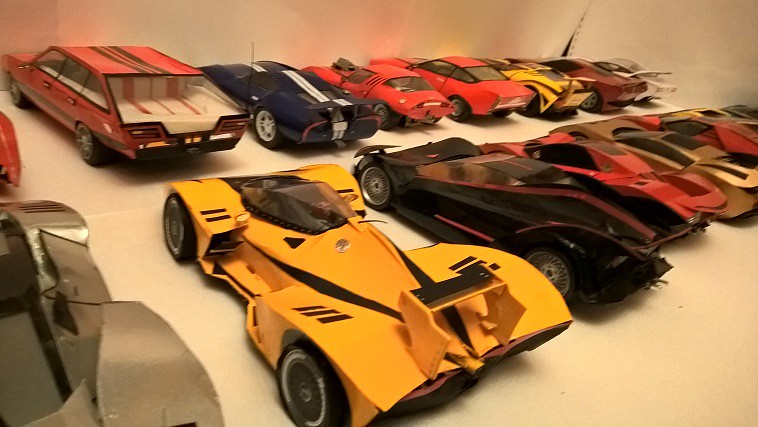The photograph features a collection of 14 meticulously arranged model cars on a white surface with a pure white background, reminiscent of a makeshift display area possibly constructed from printer paper. These cars exhibit a variety of futuristic and geometric designs, lending a somewhat artificial and prop-like appearance, as if they were crafted for movies or modeling kits. The image is taken from a slightly elevated angle, with all the cars oriented towards the top left.

There are two rows of cars, seven on each. Although the two cars on the left side are partially cut off, specific details are visible. The top row includes a red station wagon with black racing stripes closest to the cut-off edge, followed by a sequence of cars: red, black, red, red, yellow, maroon, and white. The bottom row starts with yellow, black, red, copper, red, and ends with two indistinguishable cars due to the angle.

The yellow Formula One racing car, nearly centered in the bottom row, stands out with its distinctive rear spoiler and streamlined body. The photograph’s soft orange-yellow lighting and grainy quality contribute to its aged, vintage aesthetic. Additionally, a noticeable crack in the upper right-hand corner where two pieces of paper meet further accentuates the homemade aspect of the display setting.